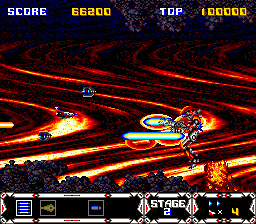A low-definition screenshot from a vintage 1980s video game, showcasing a central creature wielding what appears to be a lightsaber. The background is composed of vividly bright orange paths resembling rivers or roads. Scattered within this scene are small pieces of machinery or possibly miniature aircraft. At the top of the screen, the word "SCORE" is displayed in white, with a current score of 66,200 in yellow. To the right, the word "TOP" is followed by a high score of 100,000. At the bottom, a detailed toolbar is present; on the left side, it features a small graphic with lines and several icons. This segment also indicates "STAGE 2." On the right side of the toolbar, the number "4" is shown alongside four small items, including an icon that resembles a shoe and another that appears to be a weapon.